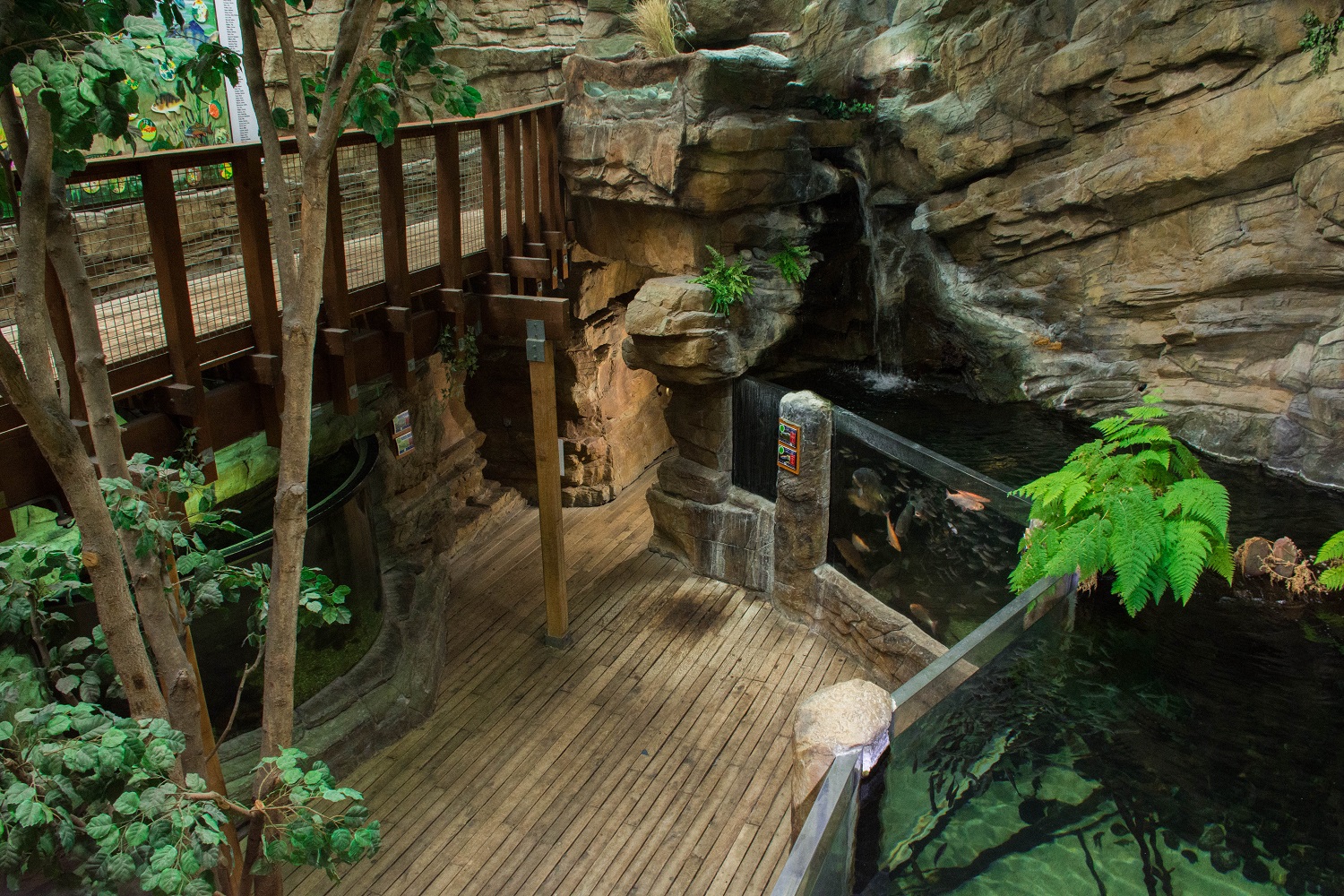The image is a detailed photograph taken inside an aquarium within a larger building. The setting features a large, open-top aquarium with greenish water, ferns, and a variety of fish in orange, brown, and white hues. Thick glass walls separate the water from the viewing area, which has a floor made of small wooden panels and a short stone wall supporting the glass. The far wall of the aquarium is designed to resemble a natural rock formation, creating an overhead extension that leads to a pathway overlooking both the aquarium and the viewing area. This pathway, visible on the upper left side of the image, includes wooden and metal railings. A thin tree with green leaves is present in the lower-left corner, adding to the scene's natural yet artificially constructed ambiance. The artificial lighting further emphasizes the interior environment of this zoolike structure.